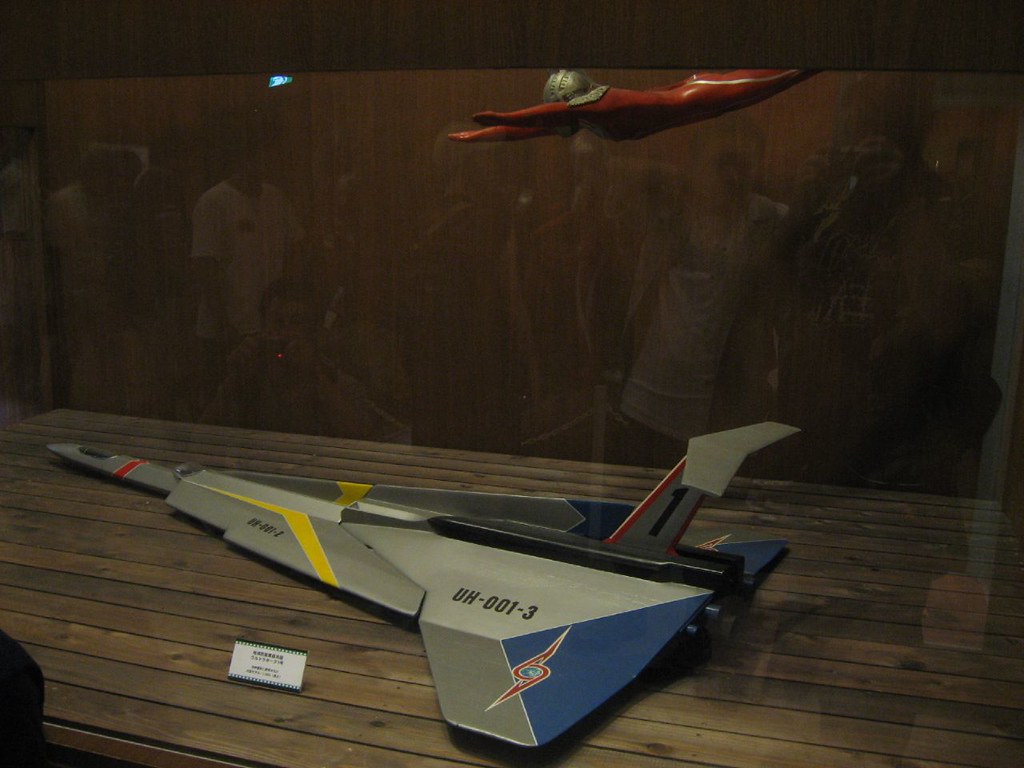The image depicts a museum display featuring a detailed and modern-looking model of a rocket ship or supersonic aircraft, encased in glass. The sleek silver model rests on a wooden plank floor and is adorned with distinct markings: a red stripe at the nose, yellow stripes along both wings, and a large blue triangle on the rear fins, with the number "1" emblazoned in black on the upright fin. Above the model, suspended along the upper part of the case, is a figure dressed in a red spandex suit with silver accents on the shoulders, wearing a silver helmet, and posed as if flying with arms outstretched, reminiscent of Superman. In front of the model sits a small, white placard featuring black text, although the details are not legible in the photograph. Reflections of the onlookers captured on the glass case add a subtle hint of human presence, enhancing the authenticity of the museum setting.